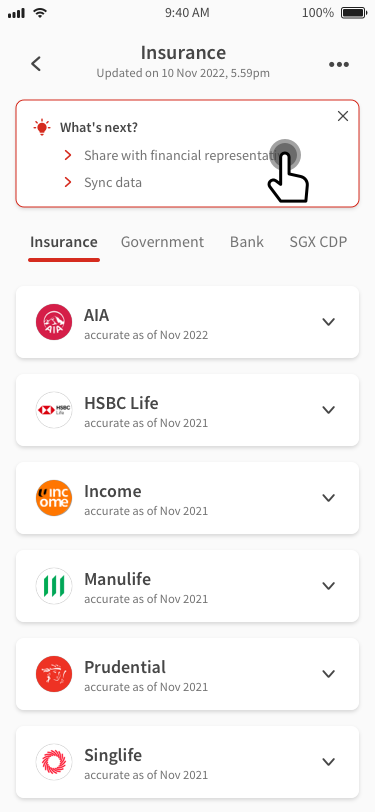Screenshot of a smartphone displaying various details and options related to insurance. The time is shown as 9:40 a.m. with a full battery at 100%. A section indicates that the insurance was last updated on November 10, 2022, at 5:59 p.m. Below this update, there is a box outlined in red featuring a red light bulb icon, with the text "What's next?" Inside the box, it provides options like "Share with financial representative" and "Sync data," with an accompanying hand icon seemingly pressing a button labeled "Insurance Government Bank HGX CDP."

Further down, there are six boxes arranged vertically, each with an arrow on the right indicating a drop-down menu, and an icon on the left representing the respective content. From top to bottom, these boxes contain the following information:

1. **AIA** - Accurate as of November 2022.
2. **HSBC Life** - Accurate as of November 2021.
3. **Income** - Accurate as of November 2021.
4. **Manulife** - Accurate as of November 2021.
5. **Prudential** - No date provided.